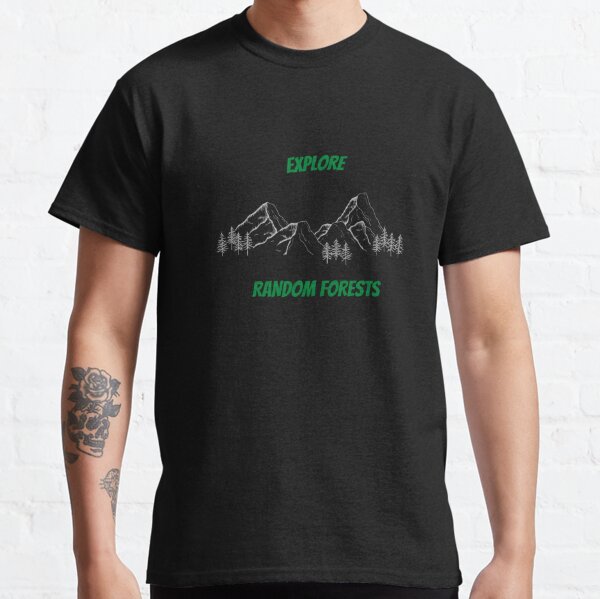The image features a close-up of a man standing against a white background. He is wearing a short-sleeved black t-shirt adorned with green text that reads "Explore Random Forests." Below the text, the shirt displays an illustration of white jagged mountains interspersed with pine trees. The image is cropped at the man's neck, so his head is not visible. 

The man has a lighter skin tone, and on his right forearm, he has a detailed tattoo of a skull with a flower above it, extending from just below his elbow and covering about five inches. The image is bright and clear, with natural lighting enhancing the visibility of the details.